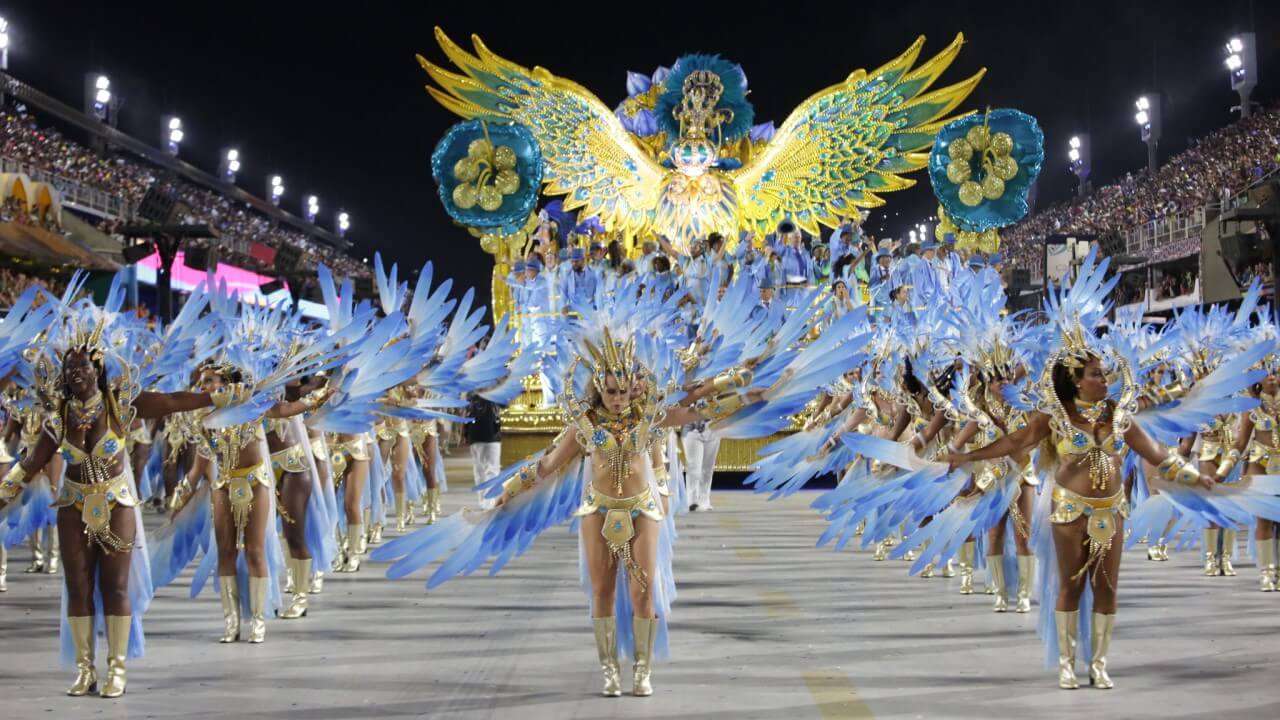The photograph captures a vibrant and elaborate nighttime event, possibly during the Olympics or a Mardi Gras celebration in Brazil. The image reveals a bustling stadium filled with spectators, illuminated by bright stadium lights. The scene unfolds on a field-like street, marked by yellow lines, where a procession of women dressed in dazzling, coordinated outfits is taking place. Each woman wears gold boots, gold skirts, and ornate brassieres that reveal their midriffs. They are adorned with intricate headdresses adorned with striking blue or periwinkle feathers, which they also hold in their hands. The women are arranged in multiple rows, performing an intricate dance or routine. Above them hovers a grand float featuring an oriental-type bird with sprawling golden and blue wings, adding to the spectacle's grandeur and festivity.